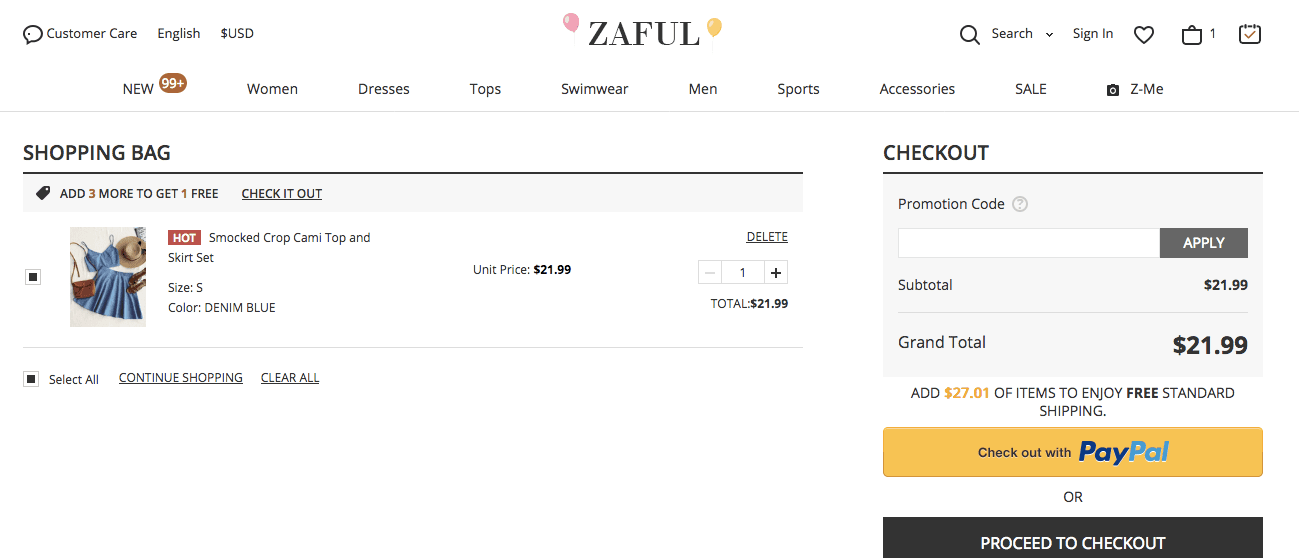This landscape-format color image is a screenshot taken from a laptop or desktop computer showing the ZAFUL website. The website's name is prominently displayed in capital letters ("ZAFUL") in black text. There are two small balloon drawings: a pink balloon to the top left of the 'Z' and a yellow balloon to the top right of the 'L'. Several navigation tabs are visible across the page, including "New" (indicating 99+ new messages or updates), "Women," "Dresses," "Tops," "Swimwear," "Men," "Sports," "Accessories," "Sale," and "Z-me." 

The site is clearly an online retail outlet specializing in clothing and accessories. The screenshot shows the shopping cart featuring one item: a smocked crop cami top and skirt set in size small priced at $21.99. The user has the option to proceed to checkout to complete the purchase.